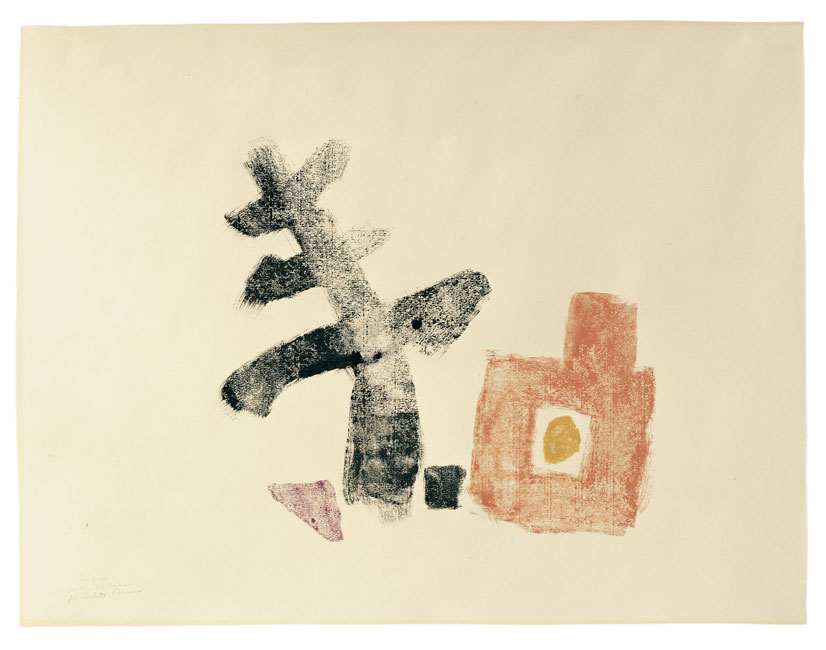The image depicts an abstract minimalist art piece set against a light beige background, with subtle variations in tone suggesting wear. In the foreground, a collection of geometrically simple forms is arranged in a sparsely populated scene, evoking elements of nature and man-made structures.

On the left side of the image, a vertical, brown stick-like form, resembling a character from the Japanese alphabet, stands prominently with three horizontal sticks intersecting it. This structure leans slightly to the left, paralleling the outline of a tree with stylized branches, small at the top and larger at the bottom, almost like a Christmas tree. Adjacent to the vertical figure is a small, dark red triangle lying on its side, adding to the composition’s abstract nature.

Towards the center-right of the canvas, a small brown box-like shape, hinted to be a house, appears. This shape includes a chimney-like protrusion at the top and an orange dot in the middle, potentially symbolizing an occupant. Nearby is a contrasting small black square, juxtaposed starkly against the warm brown tones.

Beneath these forms is a white square encasing a yellow circle, which may symbolize an egg or some focal point of energy. This arrangement offers a contrast in both color and shape, creating a focal point in the piece.

In the bottom left corner, faint three lines of handwritten text are visible, which presumably is the artist's signature, barely discernible against the worn background. The overall composition of black, white, gold, brown, and pinkish tones, rendered with what seems to be paint or pencils, evokes a mysterious and contemplative mood, reflective of an abstract, modernist style.